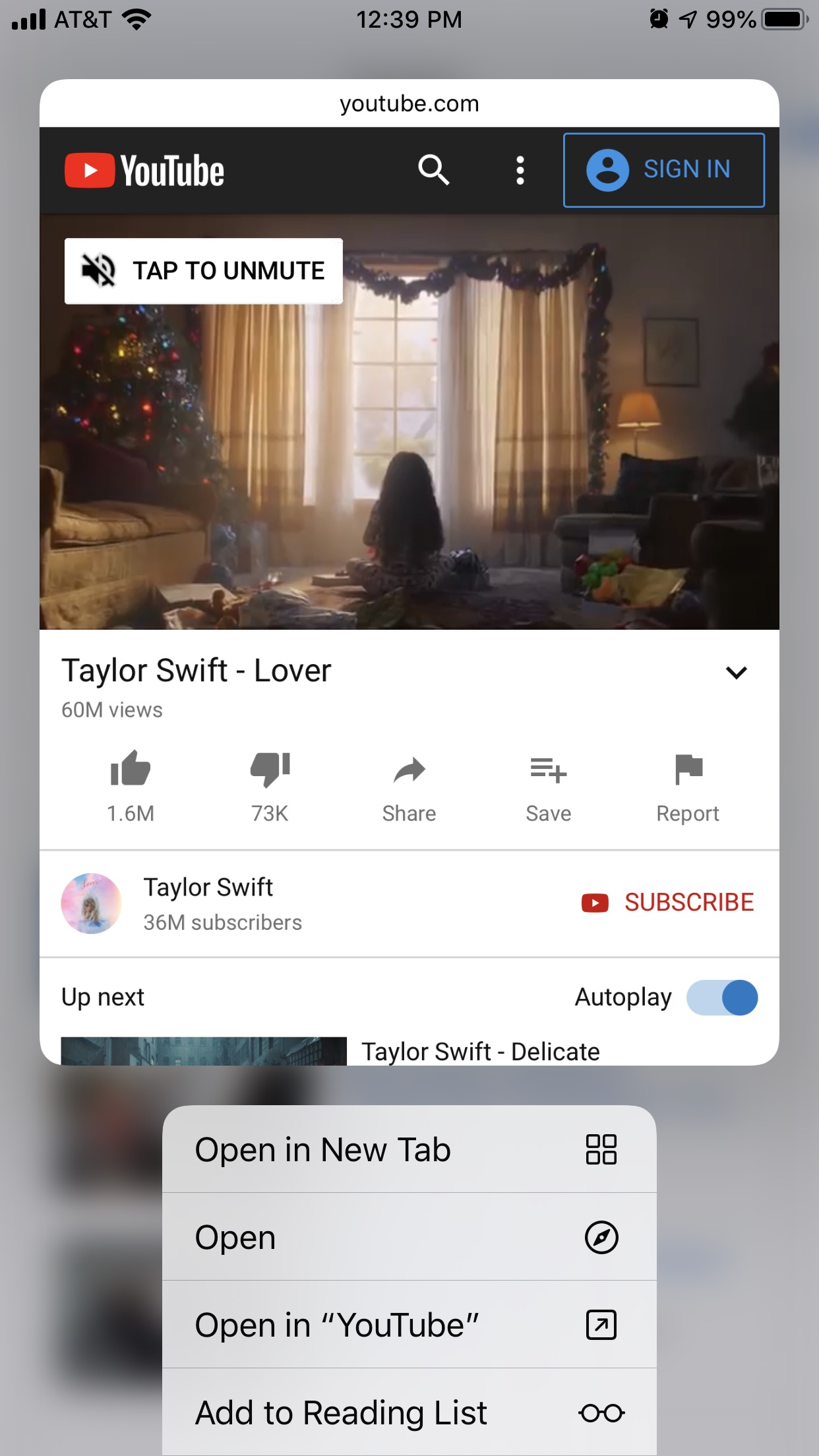The vertically rectangular image is a screenshot captured from a cell phone. The background is a gray area highlighting the phone's interface, and at the top, various status icons are displayed. On the left side, the signal bar and AT&T carrier name are visible next to the Wi-Fi icon. Centrally placed is the time, 12:39 p.m. On the right side, there are icons for an alarm and a nearly full battery at 99%.

The central focus of the screenshot is two overlapping pop-up windows. The first pop-up window belongs to YouTube.com, identified by the YouTube logo in the upper left and a "Sign in" button on the right. The featured image within this pop-up depicts a child standing near a large window, viewed from behind. The room is festively decorated with Christmas ornaments. A "Tap to unmute" button is visible in the upper left corner overlaid on the image.

Below the image, the description reads "Taylor Swift, Lover" with "60 million views" noted nearby. Icons for thumbs-up, thumbs-down, share, save, and report actions are listed below the view count. Beneath these icons, the channel "Taylor Swift" is displayed with "36 million subscribers" alongside it. A "Subscribe" button is positioned on the right.

The second pop-up window directly underneath the YouTube content is a vertical list offering several options: "Open in new tab," "Open," "Open in YouTube," and "Add to reading list."